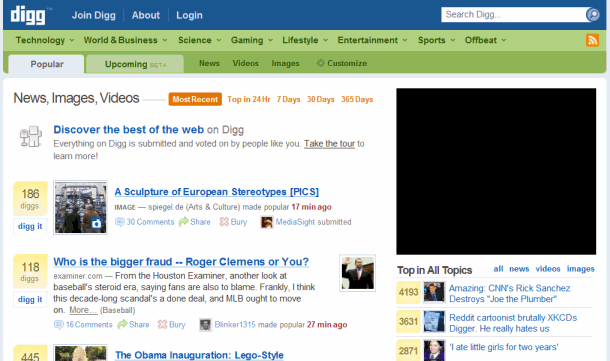This photo captures a detailed screenshot of the DIGG website, a platform that aggregates news and trending content. The image is landscape in orientation and rectangular, approximately one and a half times wider than it is tall. The overall design features a light bluish border along the left and right edges, framing the content.

At the top of the page, there is a dark blue header bar, extending across the width of the site. Inside this header, the large white letters spell out "DIGG" on the left side. Next to it, smaller white text options read "Join DIGG," "About," and "Login," followed by a white search bar positioned on the right.

Directly beneath the header, an olive-green navigation bar presents black text options and drop-down menus. These menus are labeled "Technology," "World & Business," "Science," "Gaming," "Lifestyle," "Entertainment," "Sports," and "Offbeat." On the right end of this bar, there's a recognizable orange and white RSS feed icon.

Below the olive-green navigation is a darker green section featuring white tabs labeled "Popular" and "Upcoming," with "Popular" currently highlighted with a purple font, indicating the active selection.

Further down, a white content area categorizes posts under labels "News," "Images," and "Videos" in black text, with certain elements highlighted in orange. An orange button with white text reads "Most Recent," introducing the latest articles. Below this, a series of blue hyperlinks with black descriptions are visible. Some of these links include thumbnails and are accompanied by scores inside a yellow box. Each score box displays a number followed by the word "DIGGS," indicating user interactions with the posts.